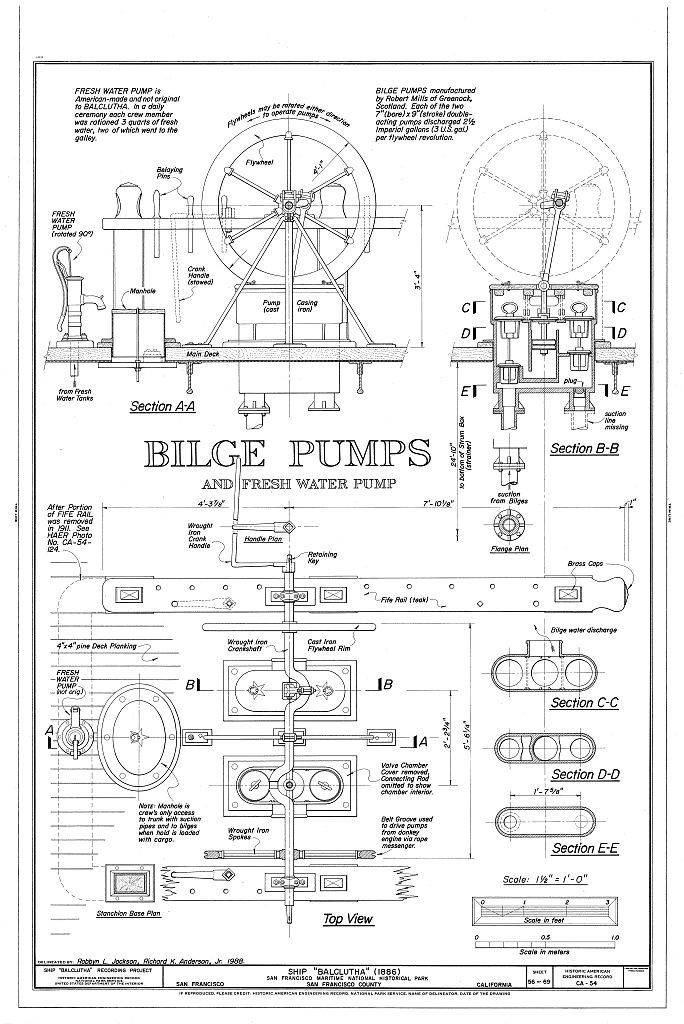This detailed blueprint-style schematic, likely drawn one to two hundred years ago and entitled "Bilge Pumps and Freshwater Pump," meticulously illustrates the mechanical design and operation of bilge and freshwater pumps. Rendered in blue and black ink on a white background, the diagram is both comprehensive and technical, displaying every aspect of the pumps, including each component's measurements and specific functions. 

The upper portion of the schematic showcases an overall view of the bilge pump, featuring a circular mechanism, alongside a freshwater pump. Detailed sectional views, labeled as CC, DD, and EE, break down the internal workings of the pumps, such as the turning rotors and internal containers, with both top and side perspectives provided to emphasize key aspects. Minutely detailed diagrams are accompanied by small text annotations that indicate the dimensions and functions of each section and part.

Additionally, the blueprint notes the historical context of the pumps, which were designed and constructed by Robert Mills, as referenced in the bottom section of the schematic. The description "Ship Balcloutha, 1886, San Francisco Maritime National Park, San Francisco County" identifies the source and era of this intricate mechanical drawing, underscoring its historical significance in maritime engineering.